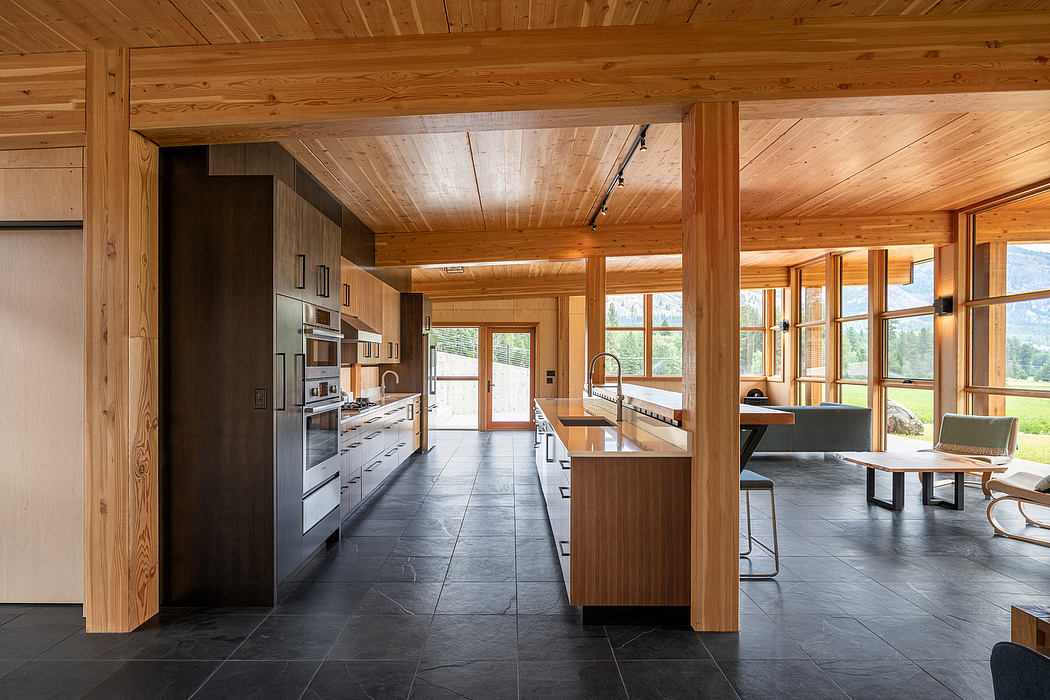The image showcases the interior of a spacious, open-plan kitchen and dining area in a house. The kitchen features a hardwood ceiling with support beams, adding a rustic charm to the space. The floor is comprised of black, stone-like tiles, lending a sleek, modern look. On the left side, there is a dark brown wooden cabinet and cupboard setup, which includes two ovens and a stovetop. Further along, there is a sink, and at the end of the setup stands a fridge. The center of the kitchen is marked by a large countertop with an additional sink, offering ample workspace.

The back wall features a large glass door framed in wood, flanked by expansive windows that offer a breathtaking view of a peaceful valley and mountains. Towards the right, near the center, there's a dining area with a low wooden table that has a distinctive bottom part, square-shaped on each end, painted black. This same side of the room boasts multiple windows, filling the space with natural light.

In the middle of the room is a boarded pillar, adding to the structural aesthetics. The ceiling is adorned with wooden beams and recessed lighting, enhancing the overall ambiance. Additionally, there are light fixtures around the ceiling, contributing to the cozy yet well-lit atmosphere. The windows on the right side also provide a serene view of a forest and an open field, making the room feel both homely and connected to nature.